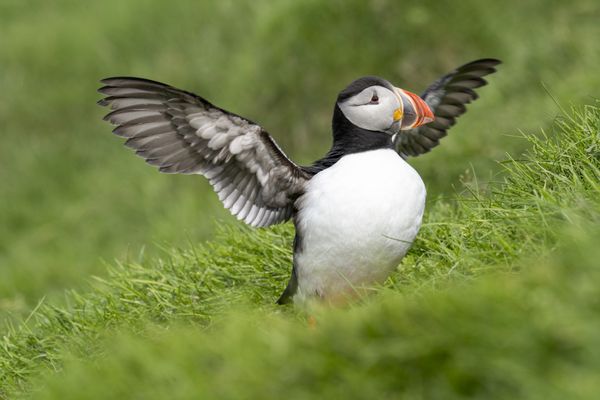A vibrant color photograph captures the stunning portrait of an Atlantic puffin, prominently set against a lush, green grassy landscape. The puffin is positioned centrally in sharp focus, with both the very foreground and background beautifully blurred, accentuating the bird's detailed features. The puffin, captured in a profile view facing right, showcases its distinctive, colorful beak, which is a striking blend of black, red, pink, orange, yellow, and gray hues. Its white breast and black upper body contrast sharply, highlighting the bird's vivid plumage. With wings fully outstretched, likely flapping as if to dry off after a dive or to soak in the sunlight, every feather on the underside is visible, adding to the intricate beauty of the scene. The puffin's legs peep out slightly, showing a hint of orange. The lush, thick grass beneath it and the overall greenery enhance the vibrant, natural setting of this captivating wildlife photograph.